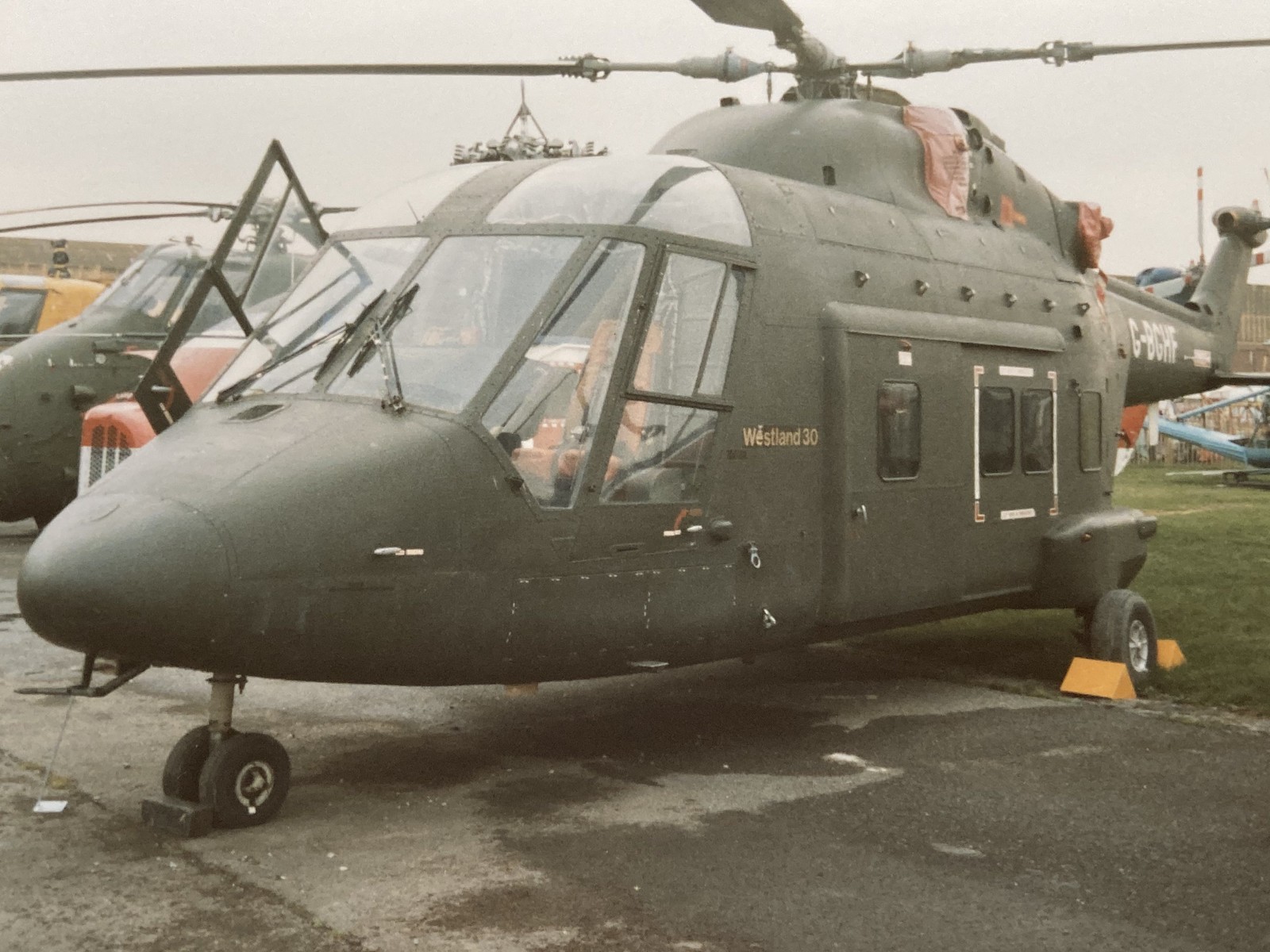In this detailed image, the scene is set outdoors on what appears to be a military base. Dominating the center are several military helicopters, prominently arranged on an asphalt road. The primary helicopter, which looks to be from the 60s or 70s, features an orange cockpit seat and is secured in place by bright yellow pyramids under its back wheel. The helicopters are painted in a greenish-gray color. Despite the overcast sky suggesting recent rain, the ground is only slightly wet.

Behind the primary helicopter is another of the same model and color. The backdrop includes a field of grass and some brick buildings, hinting at the base's infrastructure. In the background, a few people are visible, though not clearly detailed, adding a sense of scale to the scene. Among the palette of colors present—black, brown, gray, green, yellow, orange, red, maroon—the helicopter's side displays text in a yellow hue, reading "Westland 30," and the tail is marked with the code "G-BGHF." The entire setting, captured in daytime, gives a glimpse into the ambiance and environment of a military base.